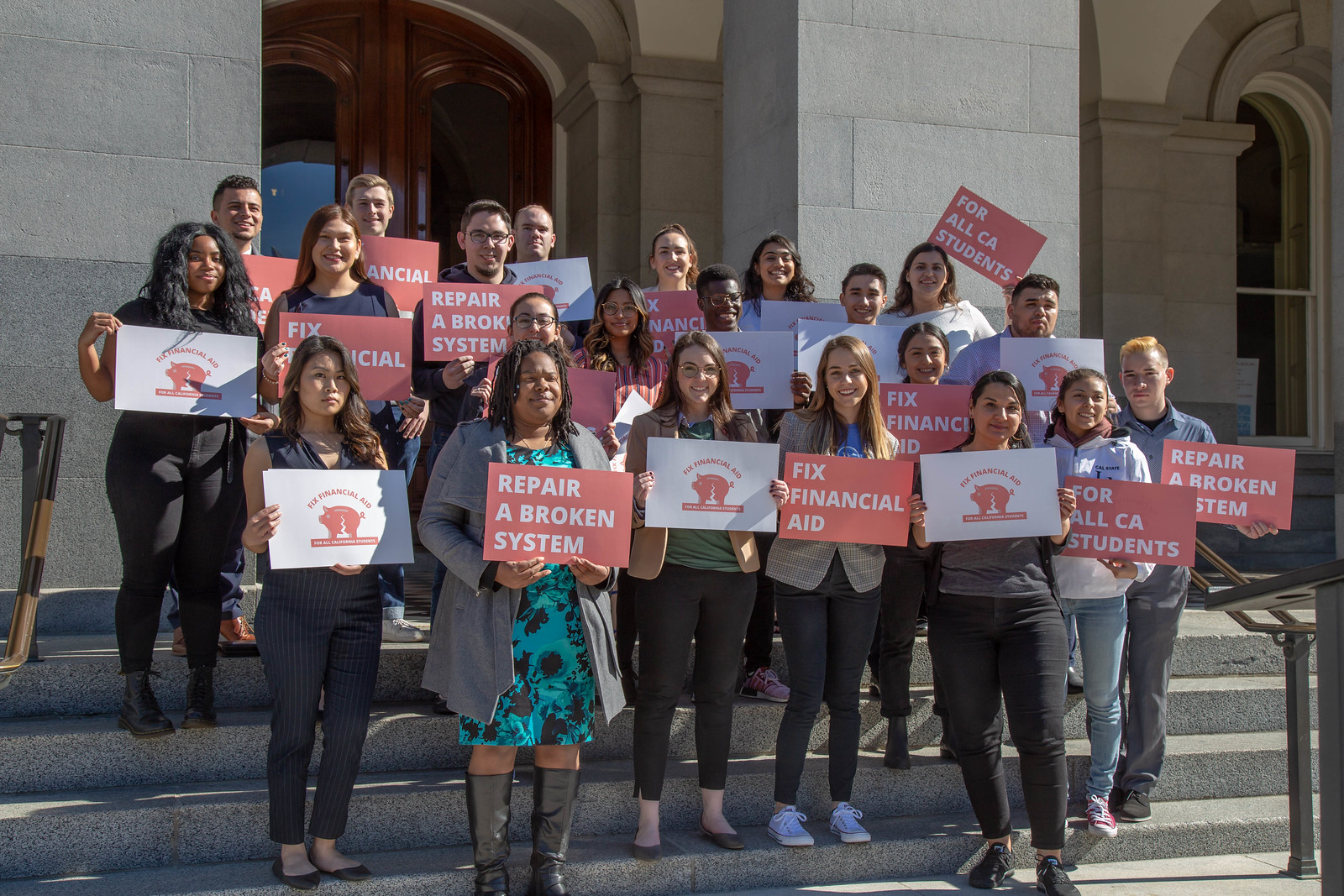This photograph depicts a diverse group of men and women standing in an orderly fashion on the steps of a gray-brick building with brown, arched doors, and white pillars, likely a school or institution. The protesters, who appear to be a mix of teachers and possibly some older students, are holding up alternating placards. The red placards with white text read "Repair a broken system" and "Fix financial aid for all California students." The white placards feature a red cracked piggy bank symbolizing financial strain, accompanied by the message "Fix financial aid." The organized display of signs highlights a protest advocating for the reform of the financial aid system to alleviate student debt and ensure better support for California students. The scene captures a range of expressions from the participants, some appearing serious and others hopeful.